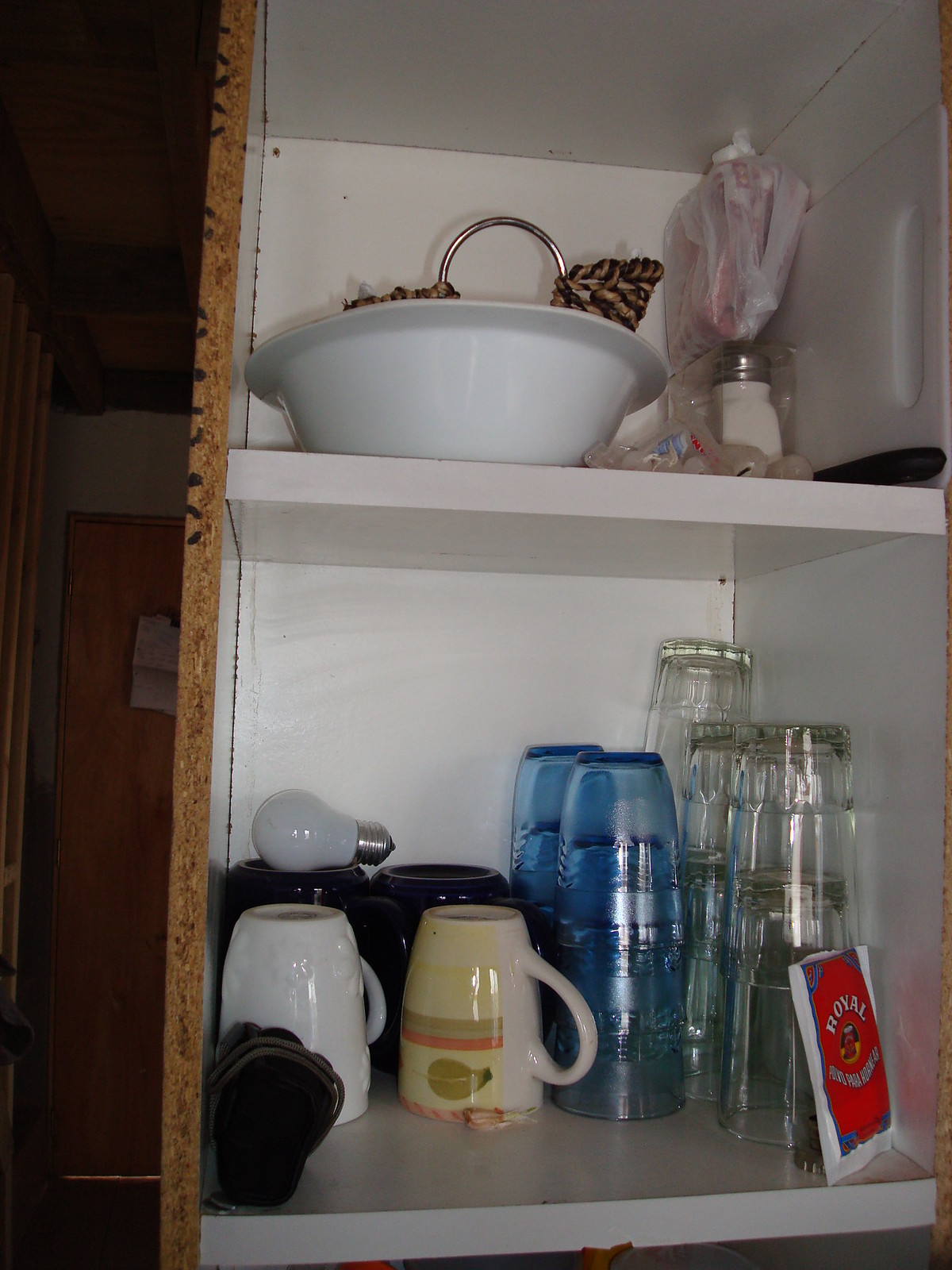The image depicts an organized cupboard with two shelves. On the top shelf, there is a large bowl filled with pine cones. Next to the bowl, there is a small jar, potentially containing salt, and a red plastic bottle with a white cap wrapped in clear plastic. The bottom shelf features a solitary light bulb, a packet labeled "Royal" that might contain a tea bag, four coffee cups, four blue transparent plastic tumblers, and approximately seven clear glass juice glasses. Among the coffee cups, two are black and situated at the back, while the front left cup is white, and the remaining cup has a leaf print in shades of yellow, orange, and green.